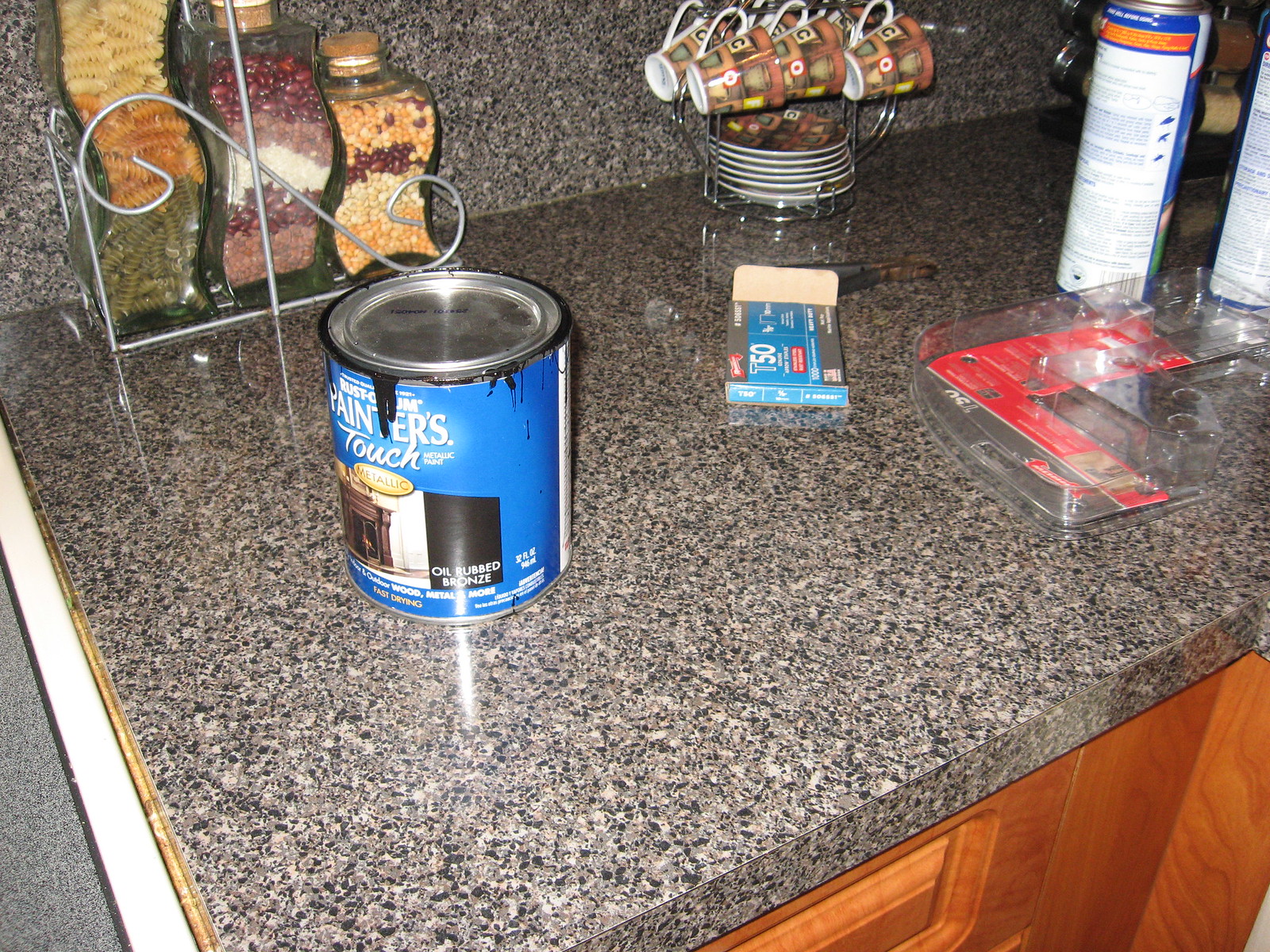A color photograph captures a close-up of a kitchen counter, which is designed to resemble granite but is actually a convincingly realistic laminate, possibly Formica or Wilsonart. The countertop features a squared-off front edge and a visible seam, distinguishing it from authentic granite. A tall backsplash runs along the back. Situated at the end of this counter, a decorative metal rack stands adorned with a trio of wavy-shaped bottles. The tallest bottle is layered with tri-colored rotini pasta in natural, tomato-red, and spinach-green hues. Beside it, a slightly shorter bottle displays layers akin to sand painting, filled with assorted beans and white rice. The shortest bottle among the trio contains dried corn and various grains, also organized in colorful layers.

To the right of these bottles is another rack, this one designed to hold crockery. The lower section cradles around six matching saucers, while the upper section, a "mug tree," suspends a set of six matching coffee mugs. Each mug features the word "coffee" amidst a brown, white, red, and yellow design, and is equipped with a white handle.

On the counter's left foreground is a can of Rust-Oleum Painter's Touch oil-rubbed bronze metallic paint, suggesting an ongoing painting project. Nearby, a box of T-50 staples lies next to an open blister pack, likely for a staple gun. Accompanying these items are two tall cylinders, presumably spray paint cans.

A glimpse of the cabinet beneath the countertop reveals a warm, medium orange-brown stain, contributing to the kitchen's inviting aesthetic.